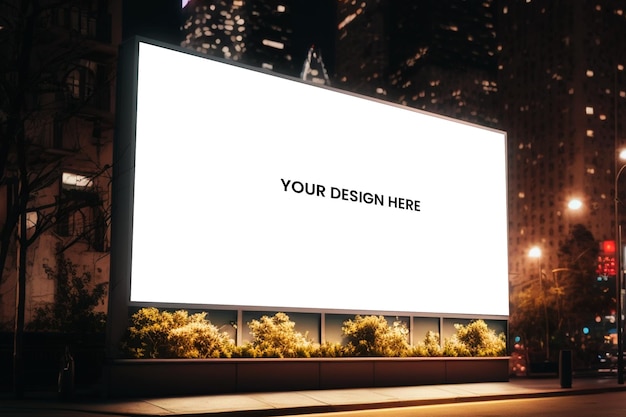The nighttime image showcases a medium-sized digital billboard situated at ground level, near a sidewalk in a large city. The billboard, lit up with a bright white screen, prominently displays the text "YOUR DESIGN HERE" in black, all-capital letters at the center. Surrounding the billboard are dark yellow bushes at its base, and the background features blurred skyscrapers with lights speckled across their facades, highlighting the urban setting. Additional streetlights and the outlines of trees are visible on both sides of the billboard, completing the cityscape scene.